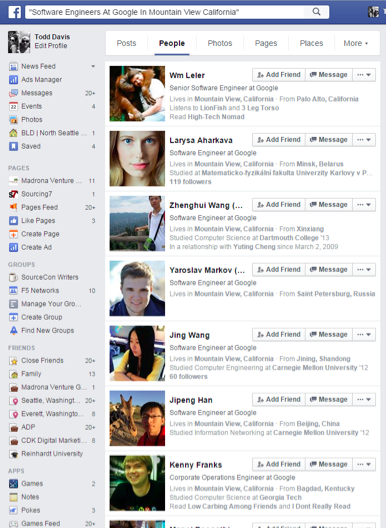A screenshot of a Facebook search results page is displayed on a computer monitor. The screen is tall and narrow, showing a search for "Software Engineers at Google in Mountain View, California." At the top of the page, navigation tabs such as Post, People, Photos, Pages, Places, and more are visible, with the "People" tab currently selected. Various search results are listed, featuring profiles of individuals connected to Google in Mountain View. 

- **Todd Davis** options to edit his profile are shown.
- **Wim Leder**, a Software Engineer at Google, has a picture that includes an enigmatic object or person on his back.
- **Larissa Arkava** appears with a close-up picture, resembling a fashion model, and is identified as a Software Engineer at Google.
- **Zwing He** (also referred to as Zwing Who or Wang) is listed as a Software Engineer at Google.
- **Yaroslav Markov** and **Jen Wang** are both labeled as Software Engineers at Google.
- **Jiping Han** continues the trend as yet another Software Engineer at Google.
- **Kenny Franks**, breaking the pattern with his name, is a Corporate Operations Engineer at Google.

All individuals are noted to be based in Mountain View, California, aligning with the search query for Google professionals in that location. The sidebar on the left of the screen shows various filter options, though the focus remains on the "People" category.